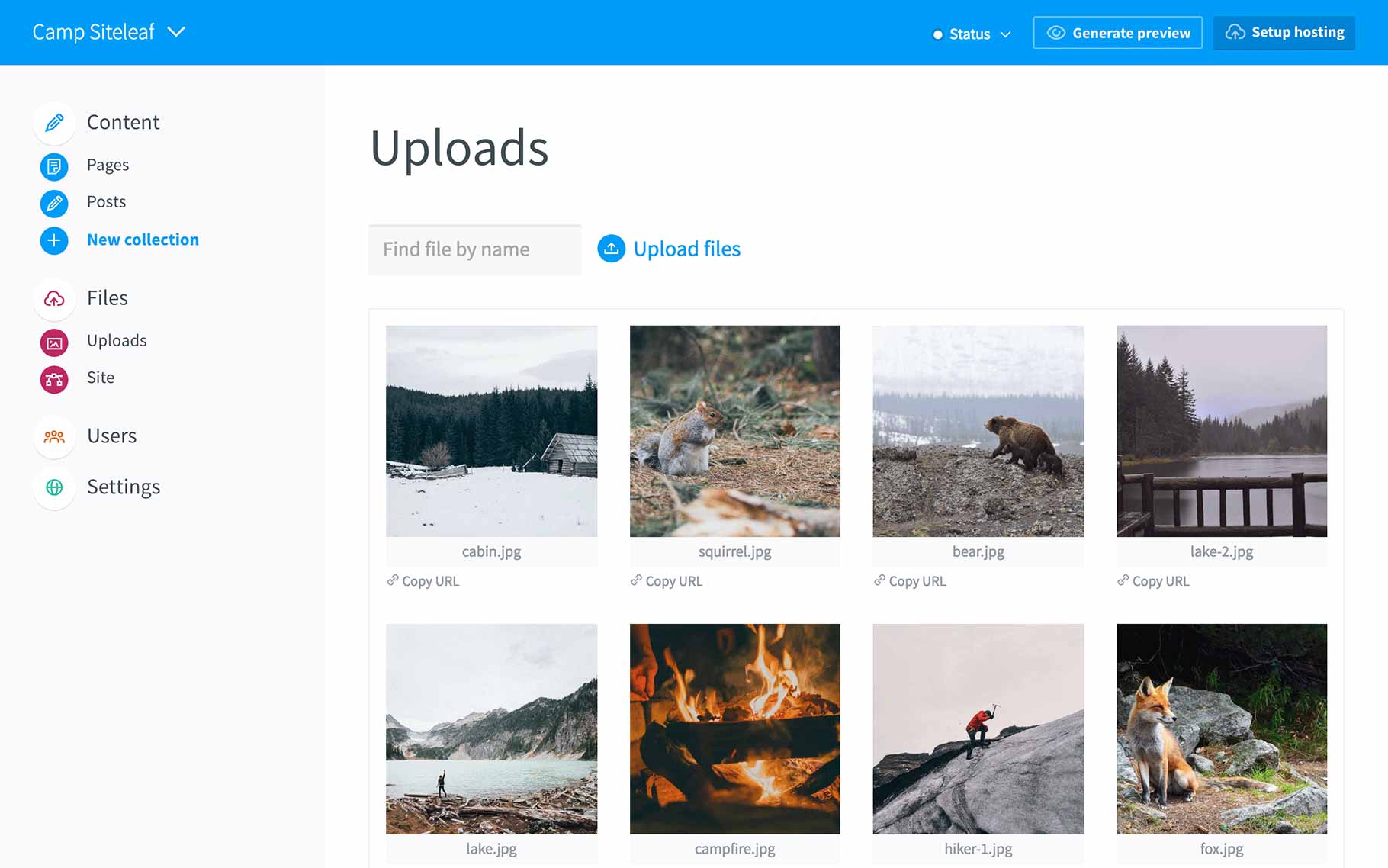The screenshot from the website "Campsite Leaf" displays a well-structured layout featuring various navigation and interaction elements. 

In the upper left corner of the site, a blue banner spans horizontally across the page, branded with the text "Campsite Leaf," and includes a drop-down menu. Over on the right side of the banner, there's a "Status" drop-down menu. Adjacent to it, there's a "Generate Preview" button, designed with a blue background, green outline, and white font. Another button labeled "Setup Hosting" is also present, highlighted by a dark blue background with a white cloud icon and white font.

The vertical navigation bar on the left side is left-justified and lists several menu options in black text: "Content," "Pages," "Posts," "New Collection," "Files," "Uploads," "Site," "User," and "Settings." The "New Collection" option stands out in blue.

The main content area of the page is focused on uploads. At the top, there is a search box with the placeholder text "Find file by name," allowing users to search for specific files. Below the search box, there is a blue button labeled "Upload Files."

Displayed below the buttons are current uploads, organized in a grid with two rows of four photographs each. Each image has its file name listed below with the option to "Copy URL" adjacent.

In the first row, the images are titled:
1. cabin.jpeg
2. squirrel.jpeg
3. bear.jpeg
4. lake-2.jpeg

In the second row, the visible images include:
1. lake.jpeg
2. campfire.jpeg
3. hiker-1.jpeg
4. fox.jpeg

The caption truncates at the bottom, with the "Copy URL" option not fully visible for the last listed image, indicating partial cut-off at the end of the displayed content.